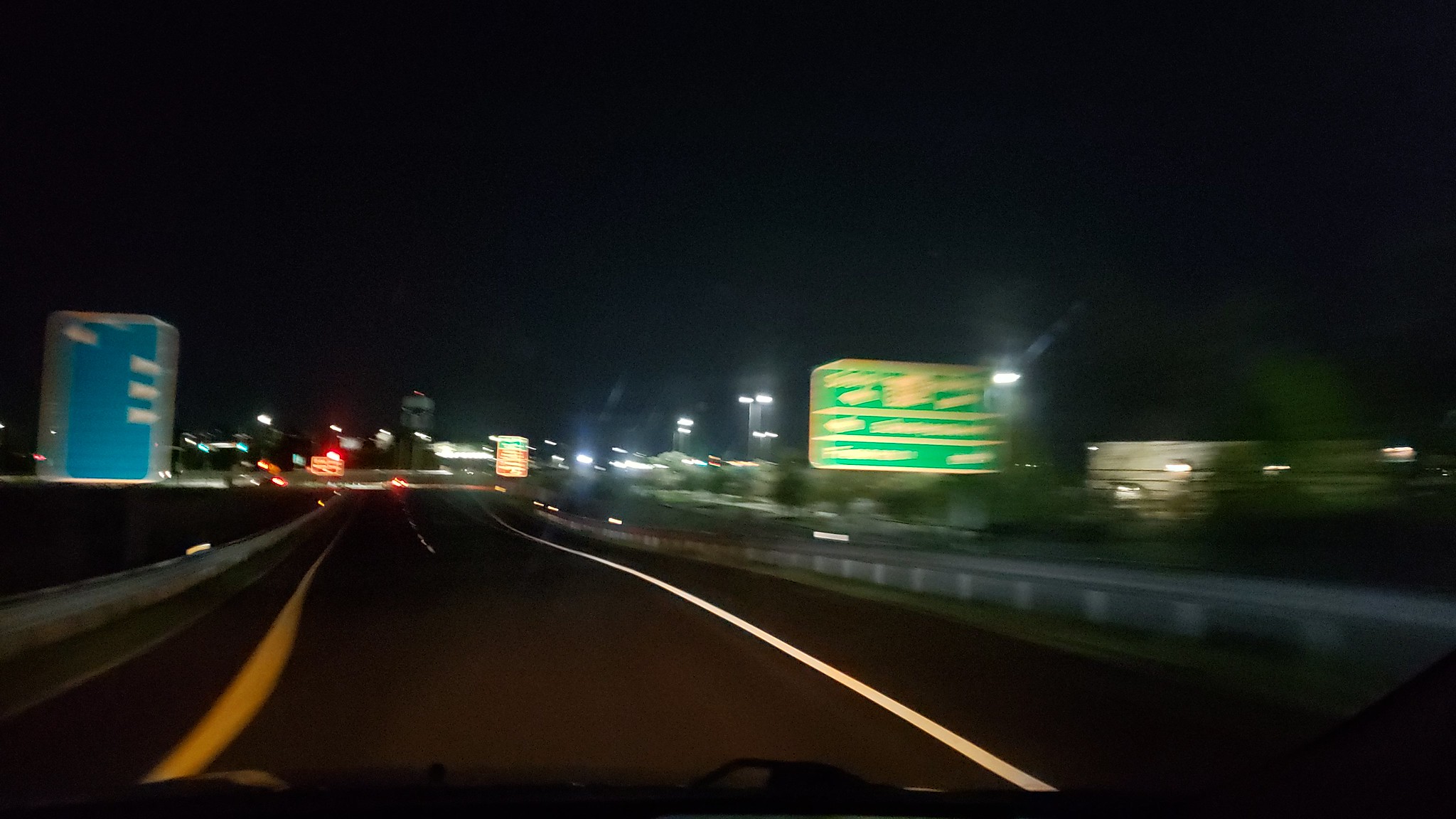A nighttime image captures a two-lane highway with a distinct white divider. The right lane appears designated for bicycles, framed by minimal light and the quiet of the night, possibly around 9 p.m. or later. Overhead is a green highway sign bearing white text, though the specifics are unreadable in the darkness. The photograph seems taken from a vehicle dashboard, potentially equipped with a GoPro, as the car heads toward a distant cityscape faintly illuminated by scattered white lights on the horizon. To the left, there's either a tall building with a bluish hue or a high truck adorned with blue cargo. At a distance, what initially seems a stoplight is revealed to be another truck, marked by a prominent red light on top.